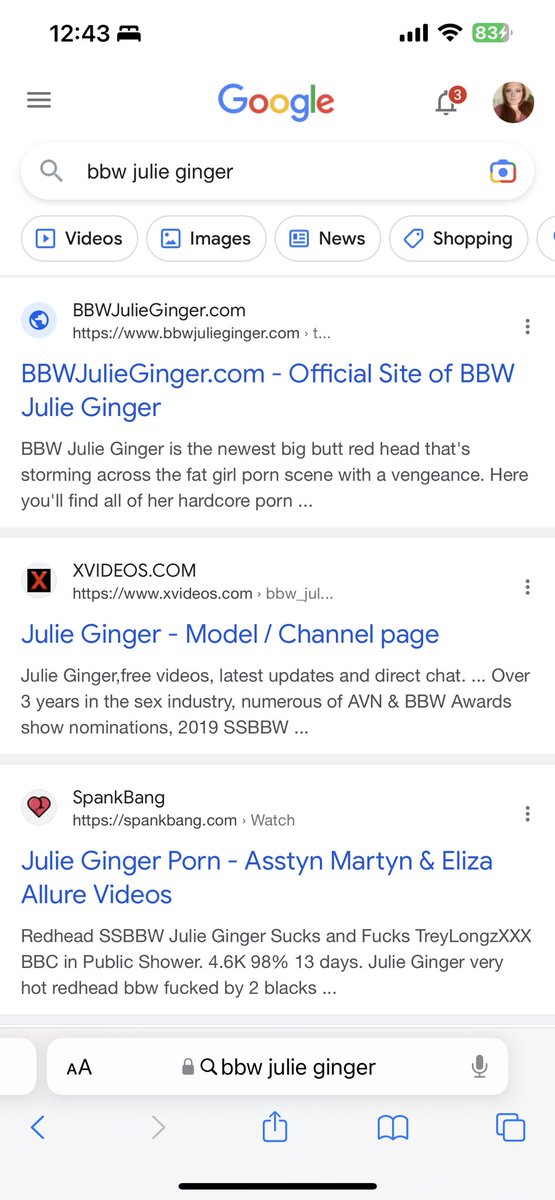This image is a screenshot taken from the Safari browser on an iPhone. The background is white, and at the very top of the screen, the status bar displays the time on the left side, a "Do Not Disturb" icon indicating Bedtime mode in the center, and icons for mobile network signal, Wi-Fi, and battery status on the right side.

The main content of the screenshot shows the Google search results page. The search query entered is "BBW Julie Ginger." It appears that this search is related to an adult film star, as the listed websites are predominantly pornographic in nature. Just below the search bar, there are small tabs for "All," "Videos," "Images," "News," and "Shopping," allowing for filtering search results by content type.

The first search result displayed is a website called "BBWJulieGinger.com." The second result is a profile page for Julie Ginger on the website "Xvideos." The third result mentions "Julie Ginger Porn" with related content on a site called "SpankBang," featuring terms like "Aston Martin" and "Eliza." 

At the bottom of the screen, the conventional Safari navigation bar is visible, showcasing buttons for back, forward, share, bookmarks, and tabs.